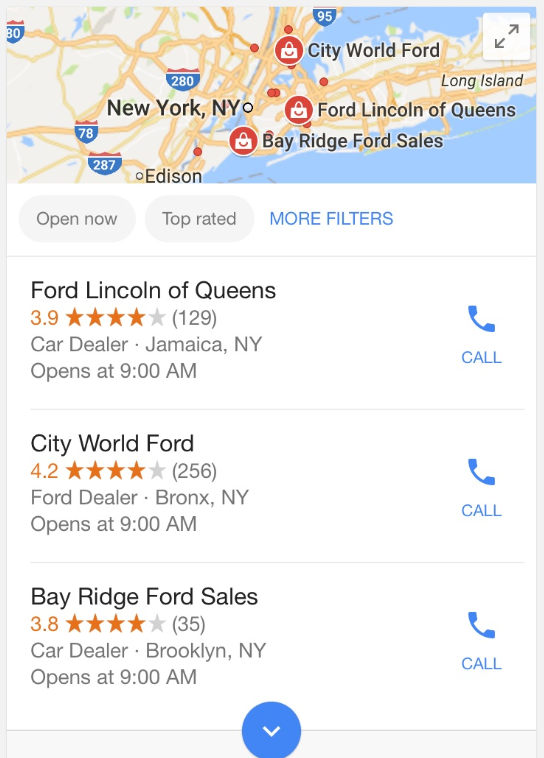A detailed caption of the given voice-described image could be:

"A Google Maps search result for Ford dealerships in the New York City area, displayed in landscape mode. The map highlights three specific dealerships: Bay Ridge Ford Sales, Ford Lincoln of Queens, and City World Ford, each marked with distinctive red pins. Additionally, several more red dots indicate other nearby Ford dealerships that are not individually highlighted. Below the map, there are filter options available, such as 'Open Now,' 'Top Rated,' and 'More Filters,' though none appear to be currently applied. The search results list shows three dealerships with ratings ranging between 3.8 to 4.2 stars. Each dealership has a call button next to its name for direct contact. At the bottom of the display, a blue button with a downward arrow suggests there are more dealerships listed that can be accessed by scrolling."